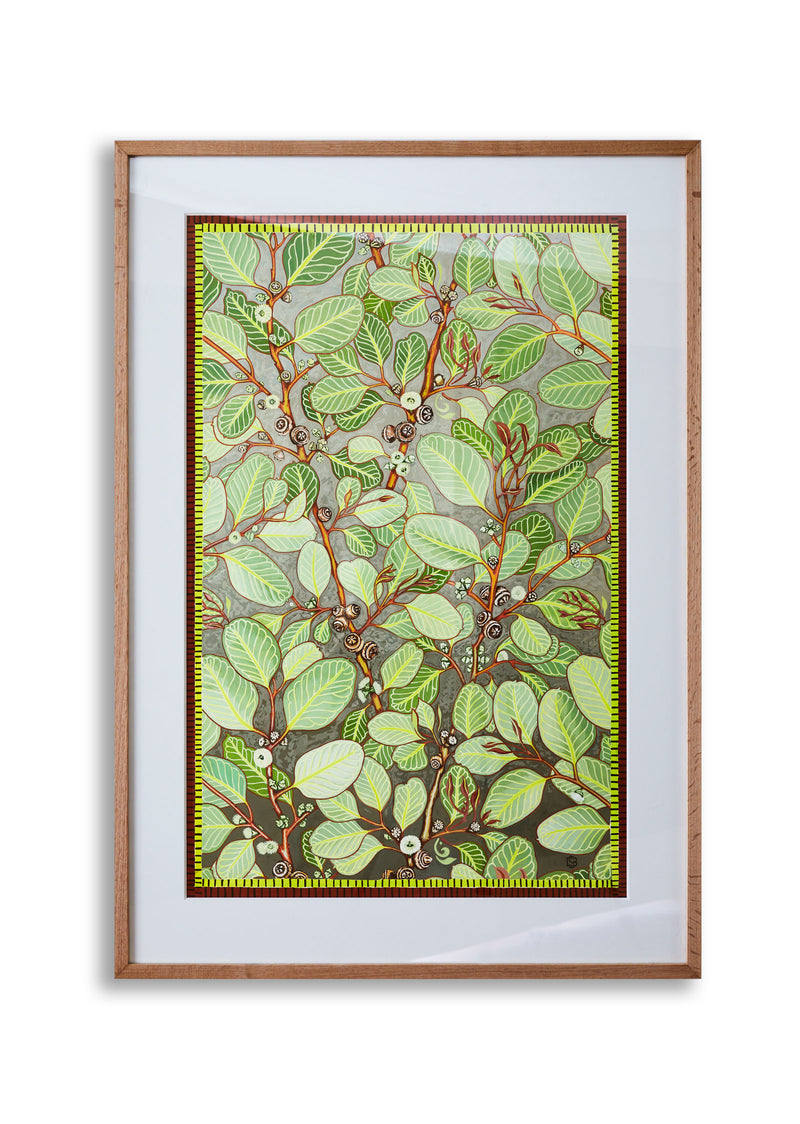This is an intricately framed and detailed painting of plant life, displayed vertically in a very thin, light-colored wooden frame. The structure is bordered with white matting, accentuating the image within. The artwork features a close-up of uniform green leaves, each detailed with a prominent main vein in yellow, from which smaller veins branch out. These leaves are attached to upward-growing branches that exhibit an orange-red hue. Amidst the foliage, small black and white nuts are interspersed. The background is a solid gray color, providing a stark contrast to the vibrant leaves and branches. Surrounding the plant imagery, there is a yellow band marked with fine black lines at regular intervals, resembling a measuring ruler, further bordered by a dark red line with similar markings, adding a unique decorative border to the painting.